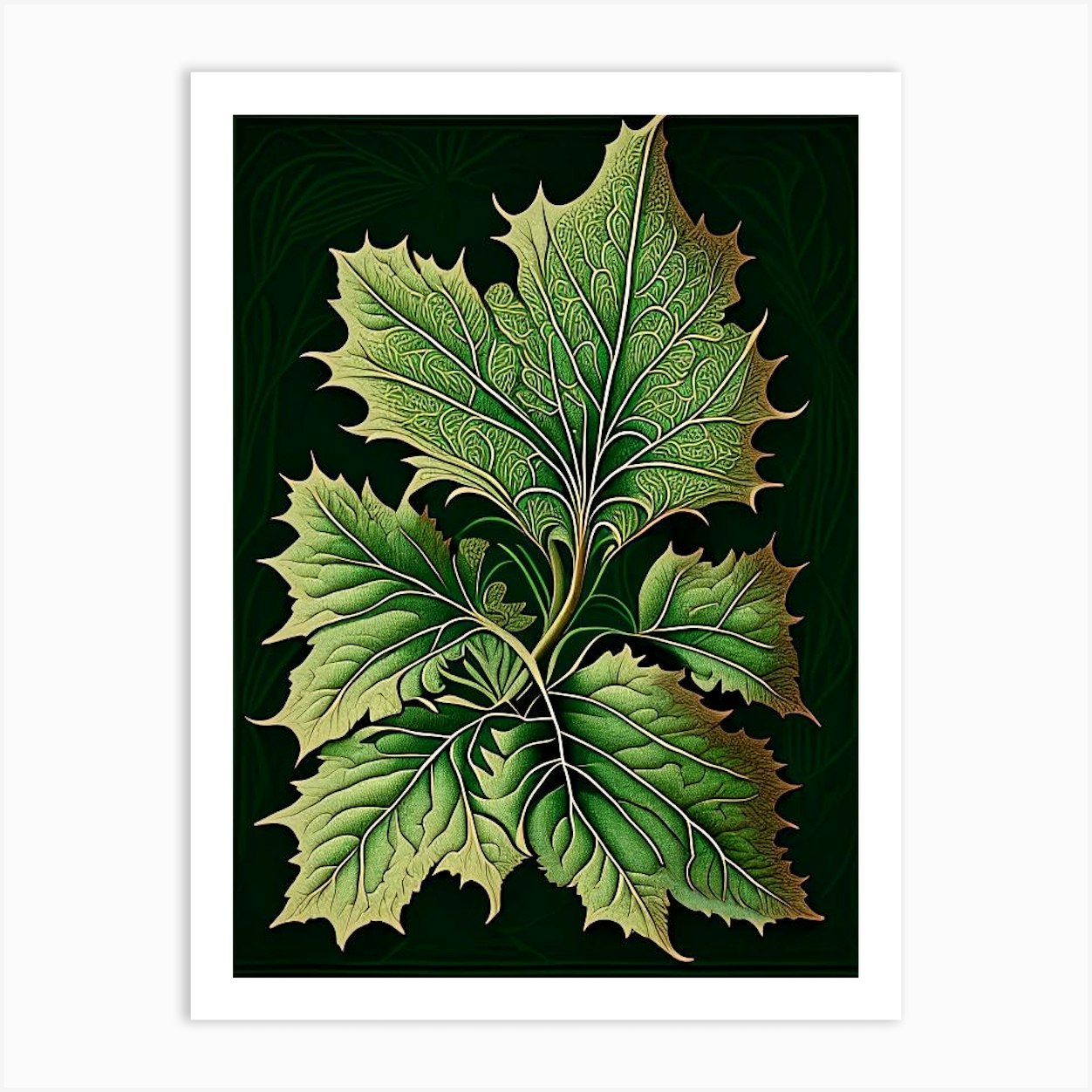The image is a vertically aligned rectangular artistic print, prominently featuring a set of green leaves on a solid black background. Encased within a white border that frames the print against a white or light gray outer background, the central image showcases several leaves, anchored to a single visible stem. The largest leaf is positioned at the top, while approximately four others fan out, with two on the sides and two or three at the bottom, some overlapping. Each leaf varies in hue from bright green at the heart to a lighter green at the edges, and they are finely detailed with veins highlighted in a gold or yellowish tint. Curved gray lines further accentuate the intricate patterns on the leaves. Despite the complexity, the image is clear and devoid of any text or signatures, capturing a bright and natural visual appeal that suggests it might be displayed in a well-lit space.